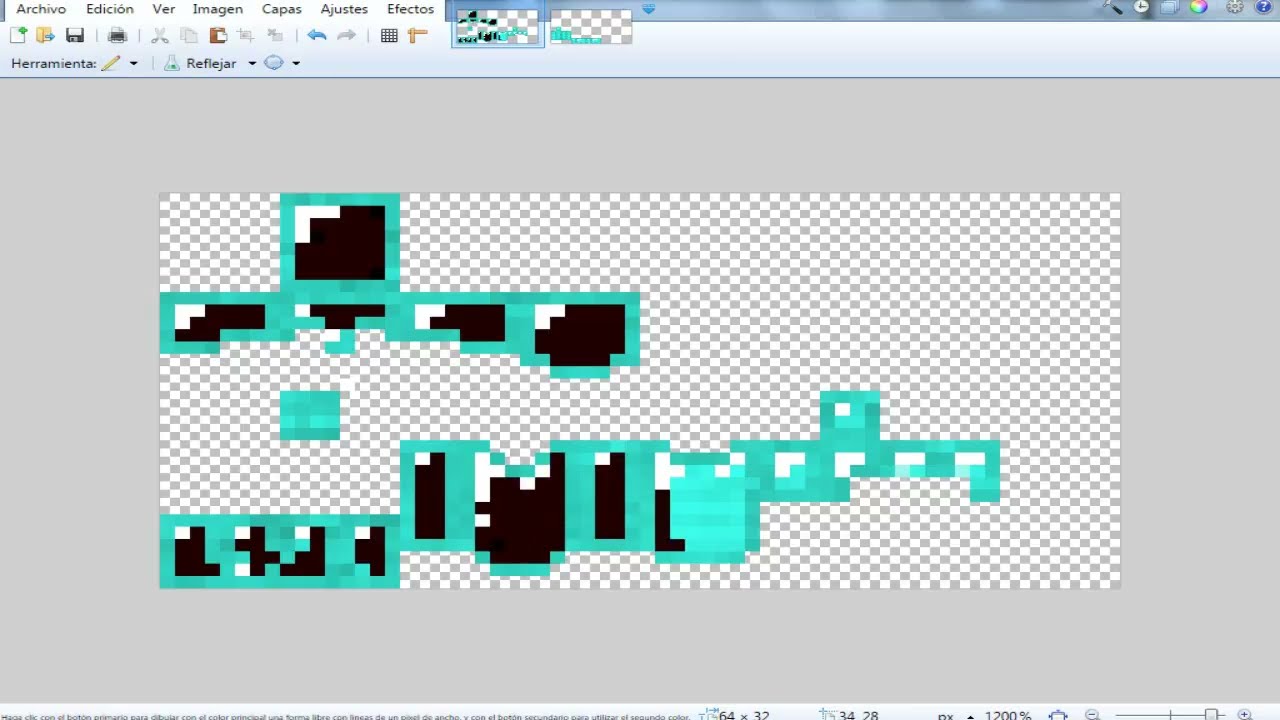The image shows a screenshot of an older graphical software interface with text in Spanish, suggesting it's a vintage or primitive program compared to modern ones. At the top of the interface, there are menu options labeled `archivo`, `edition`, `ver`, `imagen`, `capas`, `ajustes`, and `efectos`, along with tool icons such as the save disk button, print icon, cut icon, and arrows for undo and redo functions. Below these menus, the background of the computer screen appears as a solid medium gray color.

Centrally located on this gray background is a long, horizontally-aligned rectangular area featuring a small checkered pattern of gray and white squares. Overlapping this checkered area are blue (or turquoise) outlined drawings, which resemble pixelated images. Some parts of the image show black-shaded regions while others are in white. The incomplete image being created appears to contain jagged square shapes, reminiscent of an 8-bit style typically associated with old video games, possibly forming a logo. Notable in the lower part of the screen are numerics like `64x12`, `3428`, and `1200%`, indicating dimensions or zoom levels, even though some of these numbers are partially cut off. The screenshot suggests the creation process of a pixelated graphic or logo is underway.